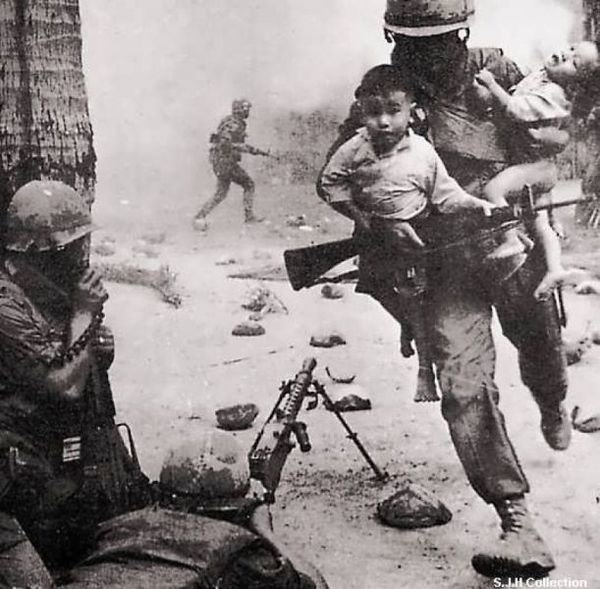In this evocative black and white wartime photograph, a soldier, clad in a helmet and dusty uniform, dashes towards safety while cradling two babies—one scarcely dressed and the other fully clothed—in his arms. The scene is fraught with tension, marked by a backdrop of thick smoke and dust indicative of recent explosions. To the soldier’s left, another uniformed figure takes cover behind a palm tree trunk, communicating through a radio. In the foreground, a man lies on the ground beside a mounted rifle or machine gun on a tripod, poised to provide covering fire. Landmines are strewn across the ground, amplifying the peril of the situation. The urgency and chaos of the scene are palpable, and the soldier’s desperate sprint underscores the raw human struggle amidst the devastation of war.